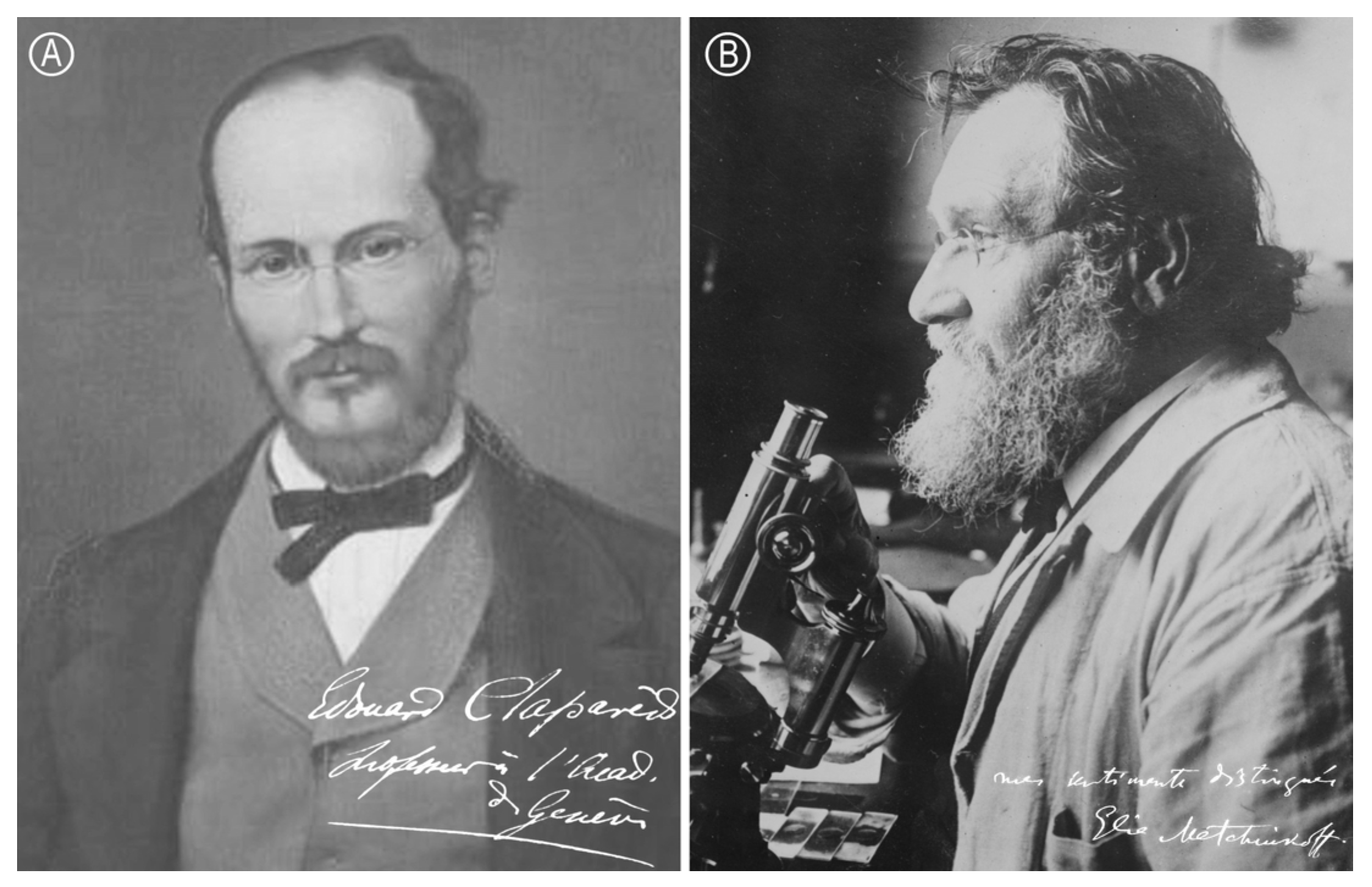The image comprises two black-and-white photographs labeled A and B, placed side by side. The photo labeled A on the left features an older gentleman with a receding hairline, spectacles, and a full beard that extends from ear to ear. He is dressed in multiple layers, including a white collared shirt, a black bow tie, a gray vest or suit jacket, and topped with a black overcoat. This image appears matted and has some writing in the bottom right, though it is not legible. The photograph labeled B on the right portrays another older man with medium-length hair and a bushy beard, viewed in left side profile. Wearing glasses and a lab coat over a collared shirt and tie, he is holding a microscope with his right hand. His pocket contains a pen, adding to the scientific ambiance. This image also features illegible writing in the bottom right corner. Both photographs exude an air of sophistication and historical significance.